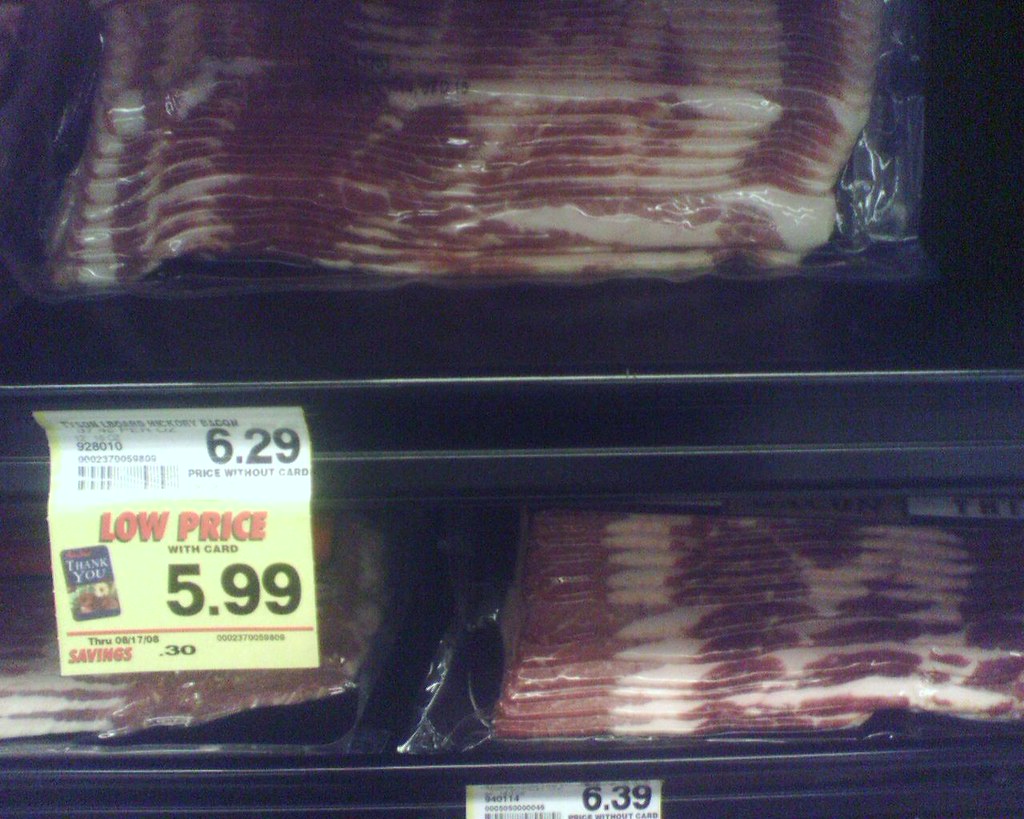The image depicts a gray, slightly fuzzy, horizontal rectangular shot of a supermarket's meat section featuring two black shelves filled with packages of bacon wrapped in transparent cellophane. The top shelf prominently displays a single package of Tyson-brand hickory smoked bacon priced at $6.29 if purchased without a card, along with a pale yellow sale tag advertising a "low price with card" of $5.99, valid through 8/17/08, and a small thank you note. In the middle of the image, barcodes and additional descriptions are partially discernible. The bottom shelf showcases two packages of Tyson dry bacon, priced at $6.39 each.